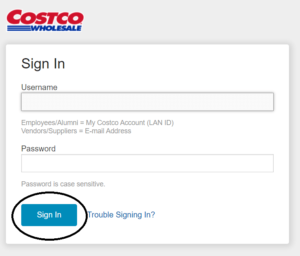The image depicts a login page for Costco Wholesale. The background is an off-white square, featuring the "Costco Wholesale" logo in the upper left corner. The Costco text is rendered in red, while "wholesale" is in blue. Directly below this, there is a white rectangle with "Sign In" indicated in the upper left corner.

Underneath "Sign In," there is a section labeled "Username," followed by a light gray input field with a darker gray outline for users to enter their username. Beneath the username field, instructions specify: "Employees/Alumni: My Costco Account (LAN ID)" and "Vendors/Suppliers: Email Address."

Following that, there is another section labeled "Password," accompanied by a similar input field with a gray outline. Below this field, there is a note stating "Password is case-sensitive." 

At the bottom of the form, on the left side, there is a blue "Sign In" button, encircled by a black line that appears to have been drawn using a photo editing tool. To the right of the "Sign In" button, there is a clickable "Trouble signing in" link in blue.

The predominant colors in the image are red, blue, white, various shades of gray, black, and hints of teal, featuring multiple shades of blue and gray for contrast.